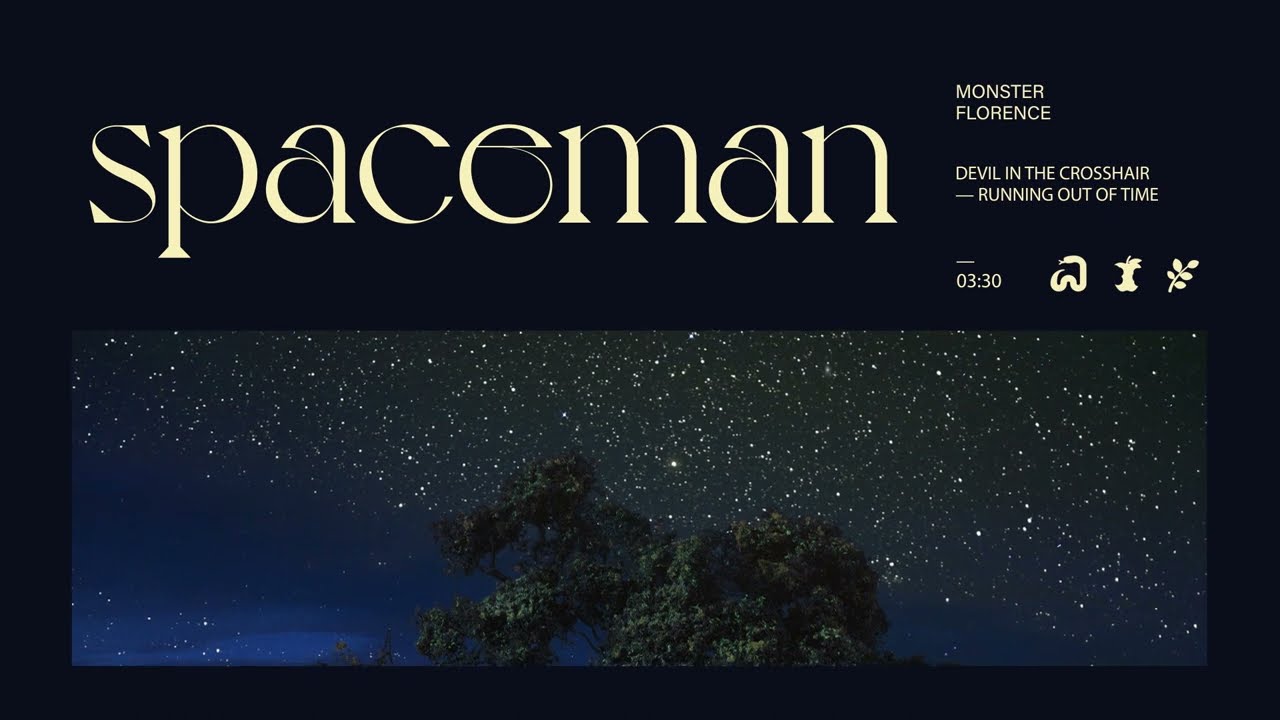The image is a wide rectangular banner with a detailed composition and a clear, layered layout. Dominating the top half is a large black triangle extending from left to right, containing white lowercase text: "spaceman." To the right, in a smaller font, are the words "monster Florence" on one line and "devil in the crosshair - running out of time" on the next line. Underneath this, there is a vertical dash and the time "03:30", indicating three minutes and thirty seconds. Adjacent to this time stamp are several symbols, including what looks like an eaten apple and a leaf, possibly representing social media or app icons.

The lower half of the image features a rich, starry night sky in varying shades of blue filled with hundreds of tiny white dots representing stars. This sky scene appears to be a finely detailed drawing or painting rather than an actual photograph. The upper part of a tree with green leaves extends into this night sky from below, adding an element of nature to the celestial backdrop. The entire image is framed within a black rectangle, suggesting that it might be part of a larger incomplete picture. The general arrangement and inclusion of timing and symbol elements hint at the image likely being an advertisement for a song or an event.